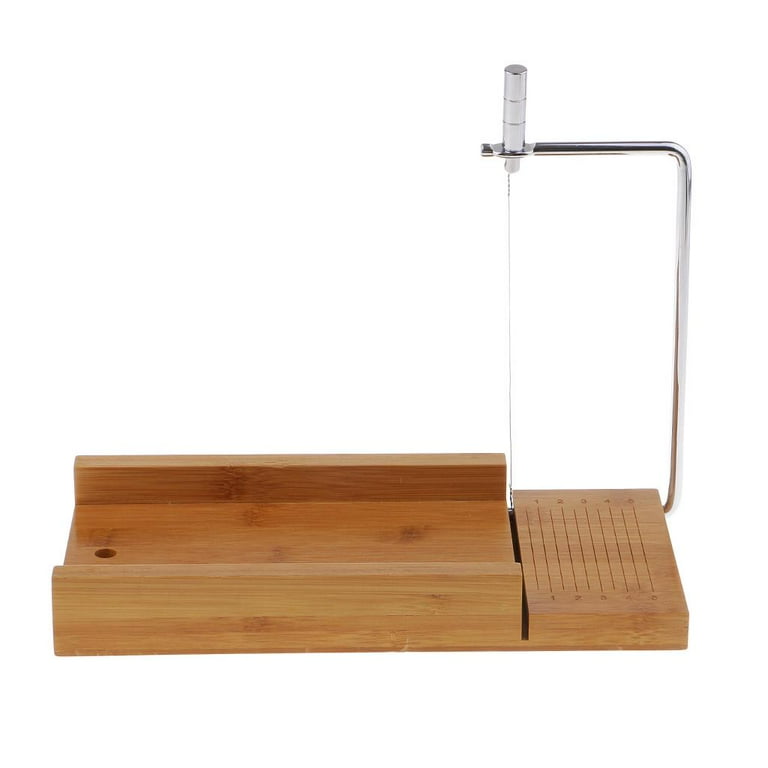This image depicts a wooden device on a plain white background, which is likely a slicer or a miter box. The base of the device is designed with a light brown wooden texture. On the left side of the base, there is a circular hole. Towards the right end, the wooden base features vertical grooves or slits. Along the top right corner, an inverted L-shaped silver metal arm extends upward and then to the left, incorporating a thin wire or blade along its left edge. This silver wire is likely used for cutting, suggesting that the device functions as a slicer for items like cheese or bread, or as a miter box for guiding a handheld saw in making straight cuts. On the right side, there is also a series of numbers, 1 through 5, etched or printed along the side of the device.